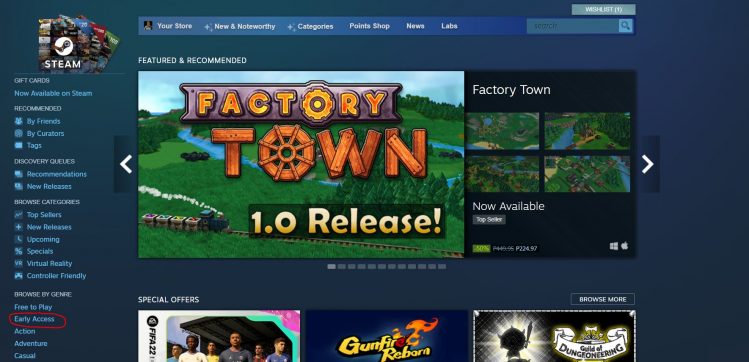The image features a screenshot of the Steam homepage. At the top, the familiar Steam logo is prominently displayed in white letters beside a circular white emblem. Below it, various navigation tabs are listed: "Your Store," "New and Noteworthy," "Categories," "Points Shop," "News," and "Labs." A blue search box is available for user queries.

On the left side, a sidebar presents multiple categories and personalized options, including a "Wishlist" indicator showing a count of one item. Additional sections provide access to gift cards, new releases, and personalized recommendations. Users can also search games by friends, curators, or specific tags.

Central to the page is the discovery area, highlighting handpicked recommendations and new releases in different genres such as "Free to Play," "Early Access" (marked with a red circle), "Action," "Adventure," and "Casual." 

A dedicated "Featured & Recommended" section highlights the game "Factory Town 1.0 Release," showcasing colorful artwork with a train running through a verdant landscape with small ponds. The game is distinguished as a top-selling title.

Further down, special offers and a "Browse More" section display diverse box art for various games, inviting deeper exploration.